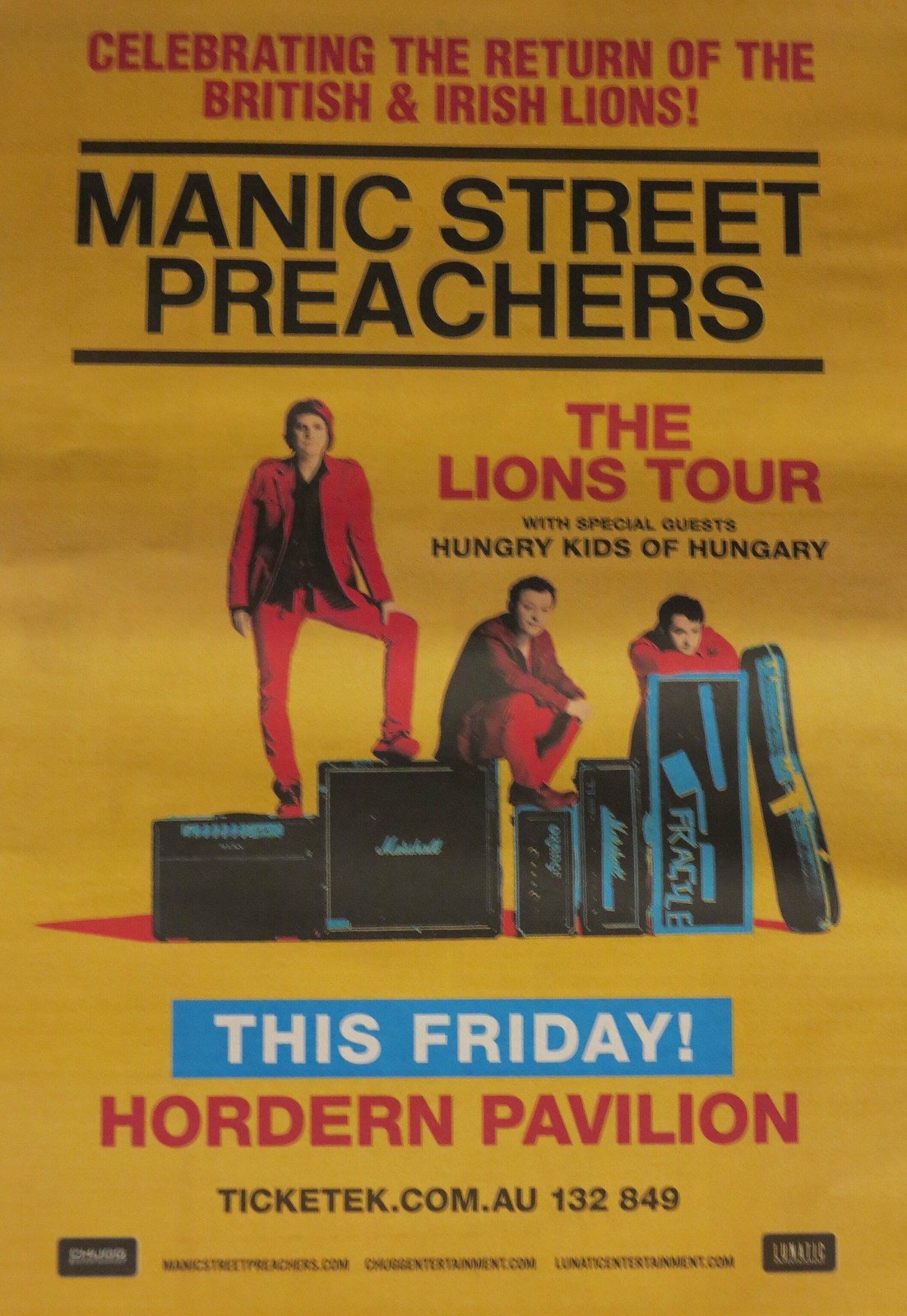The poster features a digital illustration with a goldish-yellow background, prominently advertising an upcoming concert celebration. At the top, bold red text reads "Celebrating the Return of the British and Irish Lions," with a black line separating it from the next section. Below this, "Manic Street Preachers" is underlined in black text, announcing the headline act. Underneath, in red text, it states "Underneath the Lions Tour" and "With Special Guests, Hungry Kids of Hungary."

The visual centerpiece of the poster depicts the three members of the Manic Street Preachers. The first member is sitting on top of a stack of amplifiers, his leg up with his arm resting on his knee. The second member is positioned beside him, seated on the same amp stack with his legs stretched out onto instrument cases. The third band member is hunched over, arms crossed atop another equipment container. Below this image, a blue box highlights, "This Friday," followed by red text detailing the venue, "Hoardern Pavilion." Ticket information appears as "Tickets: eku.com.au 132849," with some smaller, unreadable text at the very bottom of the poster. The color palette includes red, black, light blue, white, and dark red, emphasizing the professional and digitally crafted design.